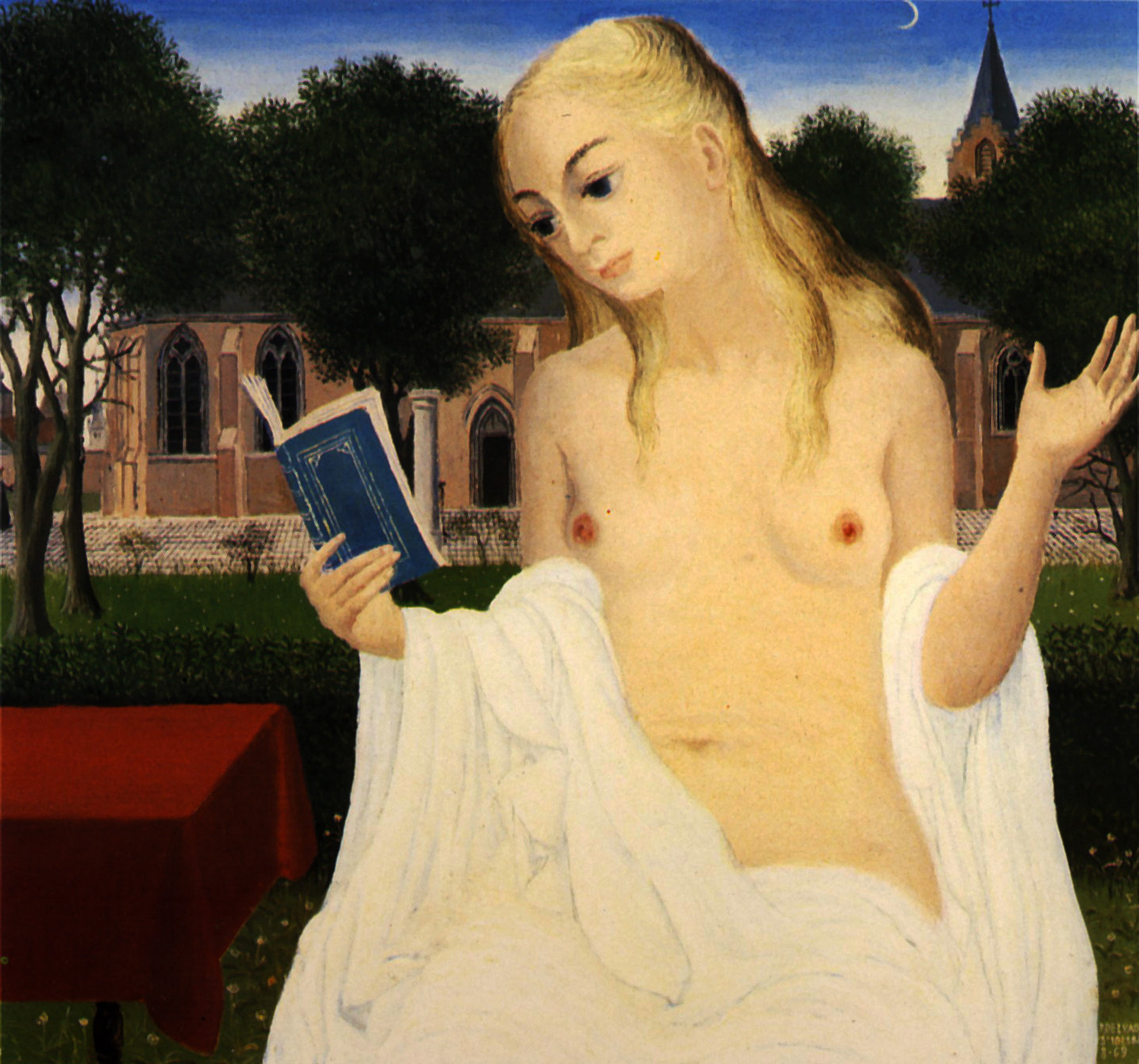In this detailed square painting set outdoors, a fair-skinned, blonde-haired woman sits nude in a garden, modestly draped from the thighs downward by a white cloth, while her bare breasts and delicate frame are exposed. Her long hair cascades down her shoulders. She thoughtfully peruses a dark blue book held in her right hand, with her left hand extended outward. In front of her is an area of lush green grass interspersed with small flowers, and to her right is a table covered by a reddish-brown cloth. Behind her stands a brick building resembling a church, complete with pointed windows, a steeple, and a noticeable cross on top, framed by four large, leafy green trees. The sky above is a deep blue, adorned by a visible crescent moon, suggesting the tranquility of twilight.